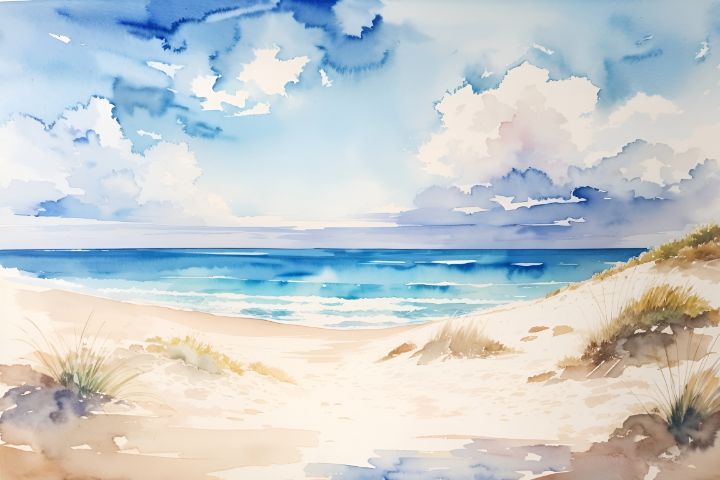This watercolor painting depicts a serene, secluded beach landscape on a clear, sunny day. The expansive sky is predominantly bright blue, dotted with fluffy white clouds, including a large one in the upper right corner. The horizon is flat, dividing the vivid sky from the ocean, which features a spectrum of blues mingling with white, indicative of the gentle waves approaching the sandy shore. The beach itself is detailed with various natural elements: patches of grass, some green and others dried to a pale yellow, along with scattered rocks. Notably absent are any people, animals, or beach paraphernalia, emphasizing the tranquility and untouched nature of the scene. The shore's terrain varies slightly, suggesting a subtle rise on the right, adding depth to the composition.